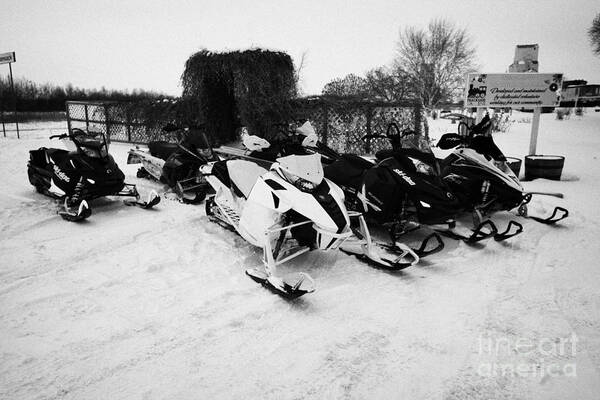The black and white photograph captures a winter scene with seven snowmobiles lined up on a snowy surface. Three snowmobiles are positioned prominently in the front: a white snowmobile with a black stripe, and to its right, two mostly black snowmobiles, one of which features white highlights. In the background to the left, four more snowmobiles can be seen, primarily dark in color. The ground is covered with snow, and a chain-link fence runs behind the row of snowmobiles. In the upper right corner of the image, a white sign with black lettering is visible but unreadable. Additionally, a row of trees and a square-shaped building can be discerned in the distant background.